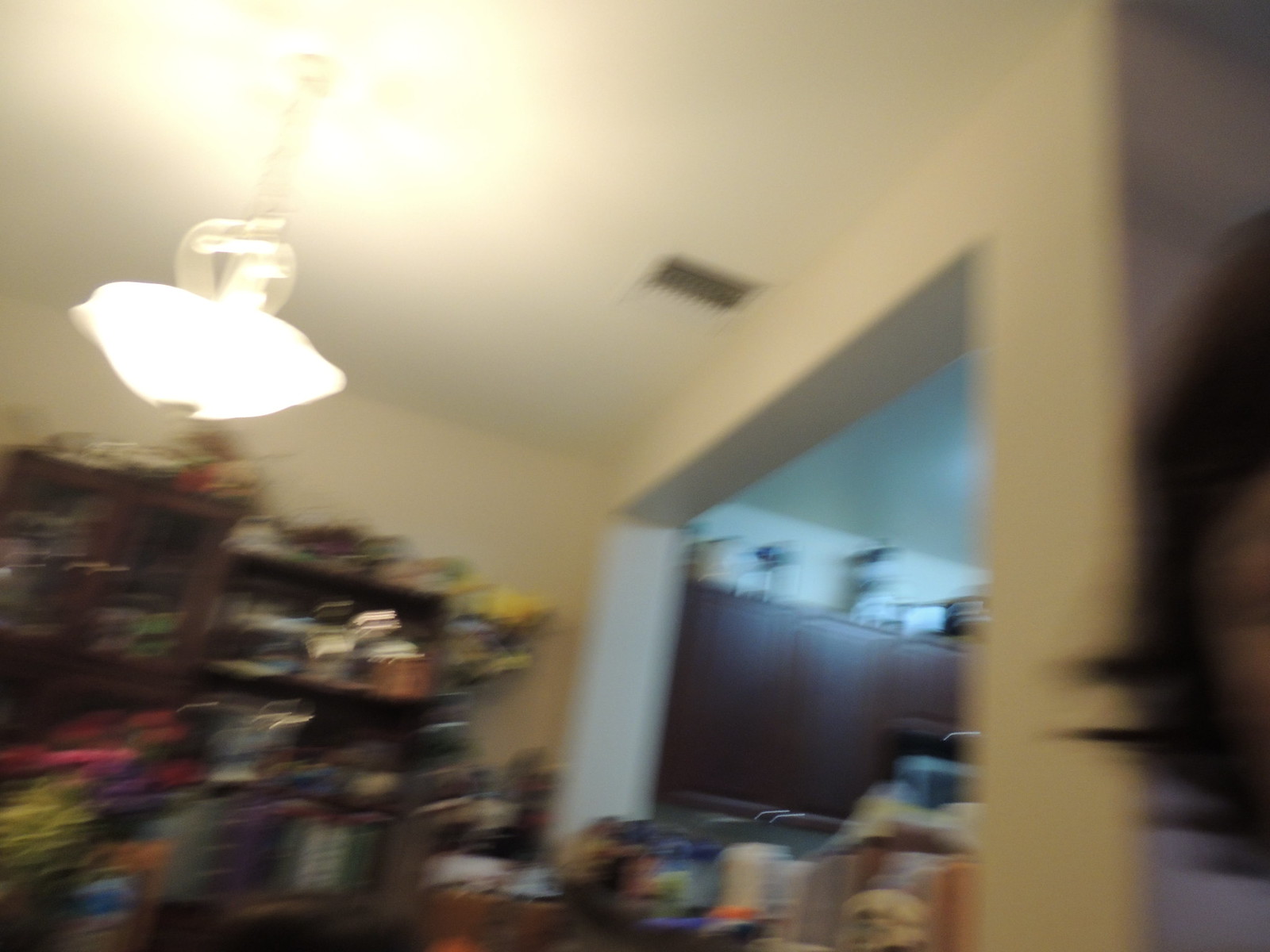In this blurry photograph, seemingly taken as a spontaneous selfie within a cluttered living space, a woman with short, dark, flared hair captures herself in front of a busy backdrop. Her partial face appears in the frame, but the focus is more on the cluttered room behind her. A light fixture on a single chain hangs from the ceiling, illuminating a space that blends into a kitchen area. The white-walled room features shelves brimming with colorful items, including dried flowers, and a dresser or bureau piled with various indistinct objects. In the right section of the photograph, dark brown kitchen cabinets are visible, with more items stored on top of them. An air-conditioning vent can be seen on the ceiling, adding to the scattered details of this densely packed interior. The photograph appears to be taken from an angle looking slightly upward, enhancing the sense of crowding and perhaps suggesting a festive decoration theme like Thanksgiving.